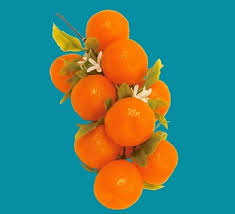This photograph depicts a cluster of small, shiny, artificial fruit resembling miniature navel oranges or possibly round berries or small tomatoes. The central focus is a group of round, orange, and slightly yellowish fruits that are tightly packed together, akin to a cluster of grapes. These fruits are set against a turquoise background, which contrasts vividly with their bright orange hue. The arrangement includes thin green stems, green leaves, and small white flowers interspersed among the fruits, giving the impression of a natural sprig. The leaves and stems are noticeably detailed, with colors that stand out against the dark and muted blue backdrop. The lighting on the artificially colored fruits highlights their glossy texture, adding to their lifelike yet slightly surreal appearance.